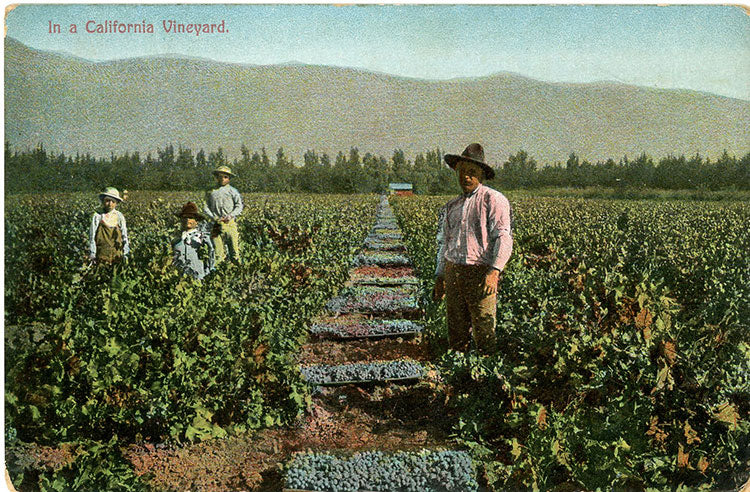This is a horizontally oriented photograph that resembles a vintage postcard from the early 20th century, characterized by its grainy, lower-quality, full-color aesthetic. The top left corner features red lettering that reads, "In a California vineyard." The scene captures a California vineyard with lush green plants and a picturesque mountain range under a clear blue sky in the background. To the center right stands a man in a black hat, white or reddish shirt (possibly stained), and green or tan pants, looking directly at the camera. Closer inspection reveals three additional figures to the left, dressed in outfits typical of farmers decades ago, including hats and simple shirts. They appear somber and are standing among bushels of grapes. The foreground consists of the vineyard's walking path flanked by rows of grapevines, suggesting a mid-20th century farming scenario. A small house and several trees are also visible in the background, enhancing the postcard-like quality of this nostalgic depiction of agricultural life in California.